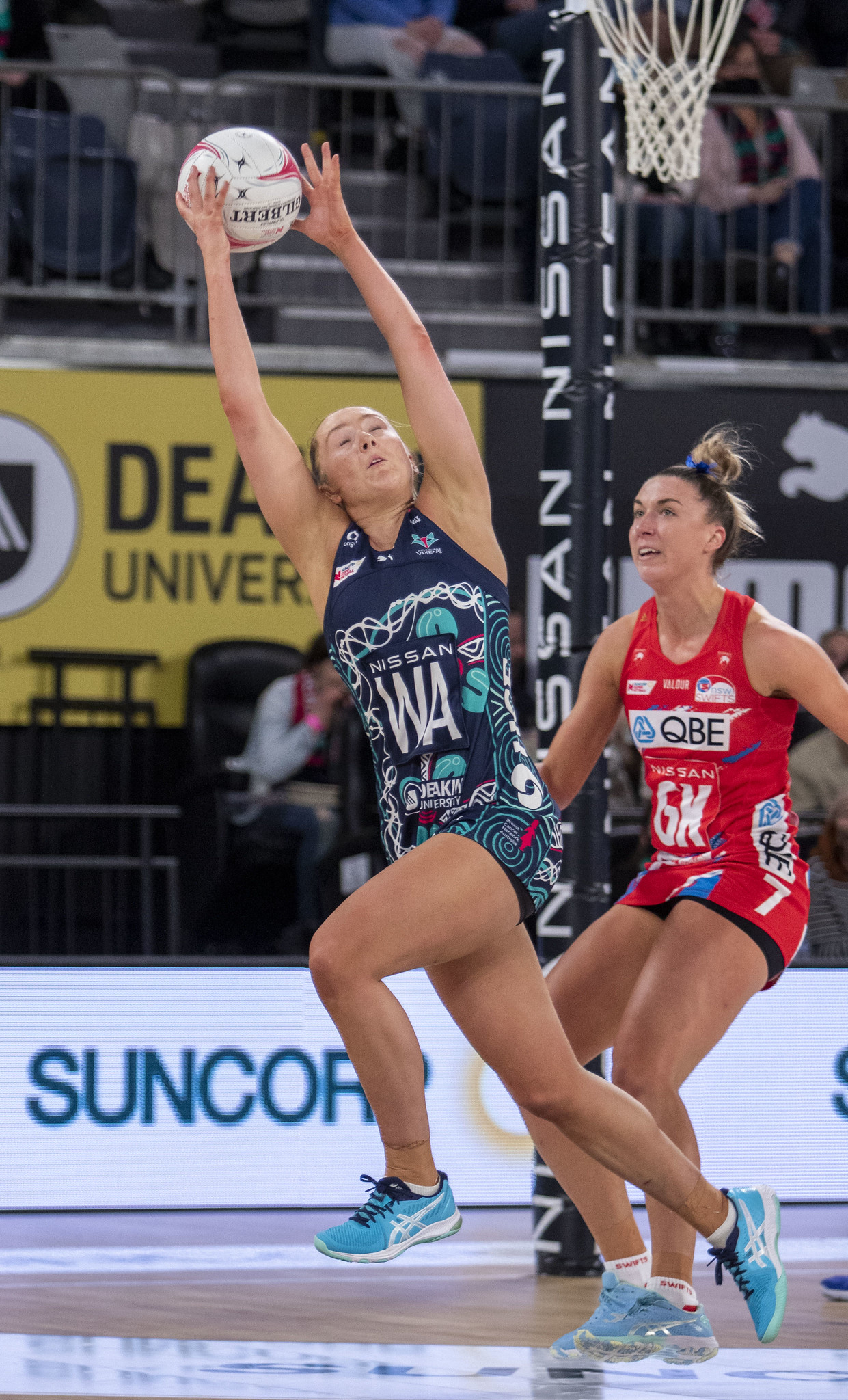The photograph depicts an intense moment with two female volleyball players in action, set in an indoor gymnasium. The player on the left, front and center, is captured leaping at an angle with her arms stretched above her head, in an attempt to catch or spike a white volleyball adorned with red and black trim. She is dressed in a dark blue tank top and shorts, emblazoned with the Nissan WA logo, and is sporting light blue tennis shoes. The athlete on the right, partially behind her, is seen in a vibrant red tank top and shorts with GH written on the front, and she also wears light blue tennis shoes. Both women appear to be in their 20s, with the one in red having blonde hair tied up. The gymnasium is identifiable by the basketball hoop in the background, mounted on a black post marked with the Nissan logo. Surrounding the court are various advertising banners in white, yellow, and black, including brands like Suncorp and Puma. The spectators are visible across an upper and lower level, adding to the dynamic atmosphere of the scene. The image, in portrait orientation, captures a moment of high athleticism and concentration, characteristic of a freeze-frame from a video.